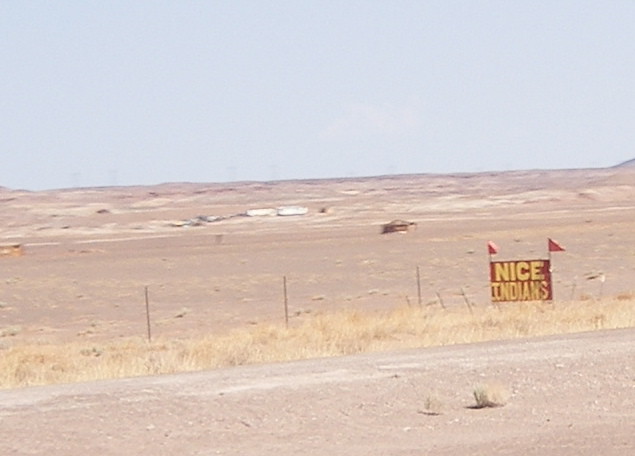This photograph captures a barren desert landscape characterized by vast expanses of sand interspersed with patches of dry, brown grass. Intricately positioned in the foreground, a segment of a fence guides the eye towards a red sign adorned with yellow text that reads "Nice Indians." Adding to the visual interest, two vibrant red flags are affixed atop the sign, fluttering subtly in the daytime breeze. In the mid-ground, a weathered brown structure stands, its details softened by distance, accompanied by two indistinct white objects further back, hinting at human presence or activity. The ground displays various clumps of sand and dirt, contributing to the scene's arid, desolate aesthetic. The entire composition is bathed in the soft, natural light of a pale blue daytime sky, completing the desolate yet captivating desert tableau.